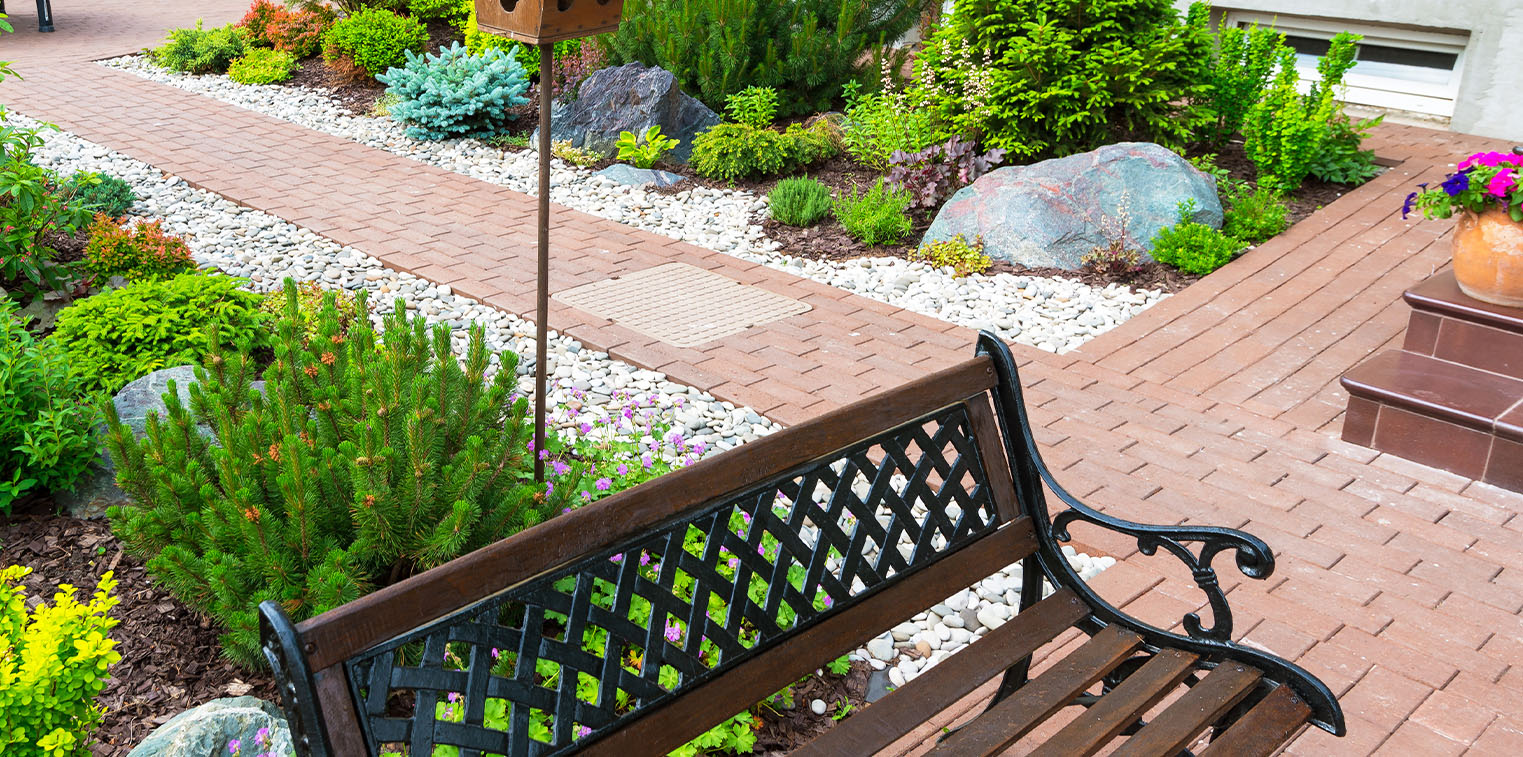This photograph showcases a meticulously maintained garden patio area, possibly a residential garden or an exhibition garden. Central to the image is a bench with wooden slats for the seat and backrest, which features a crisscross metal lattice design. The bench has sturdy wrought iron arms and legs, embodying a blend of classic and rustic styles. In front of the bench, a brick red walkway draws the eye through the space, flanked by areas of white gravel stones and neatly lined with decorative large rocks.

On the left side of the image, two steps made of reddish-brown tile, adorned with a vibrant orange planter containing pink and blue flowers, mark the entrance to the walkway. This pathway winds through a beautifully landscaped area filled with an array of colorful plants and flowers, including greens, blues, light blues, pinks, oranges, yellows, and purples. These plants vary in height, adding layers of visual interest to the scene.

Visible in the background, a tall metal pole supports a small wooden birdhouse, inviting avian visitors to the garden. To the left, the exterior of a house peeks into the frame, showcasing a gray wall and a white rectangular basement window, subtly grounding the scene in a residential setting. This detailed garden not only demonstrates a high level of horticultural skill but also provides a tranquil retreat for relaxation and nature enjoyment.